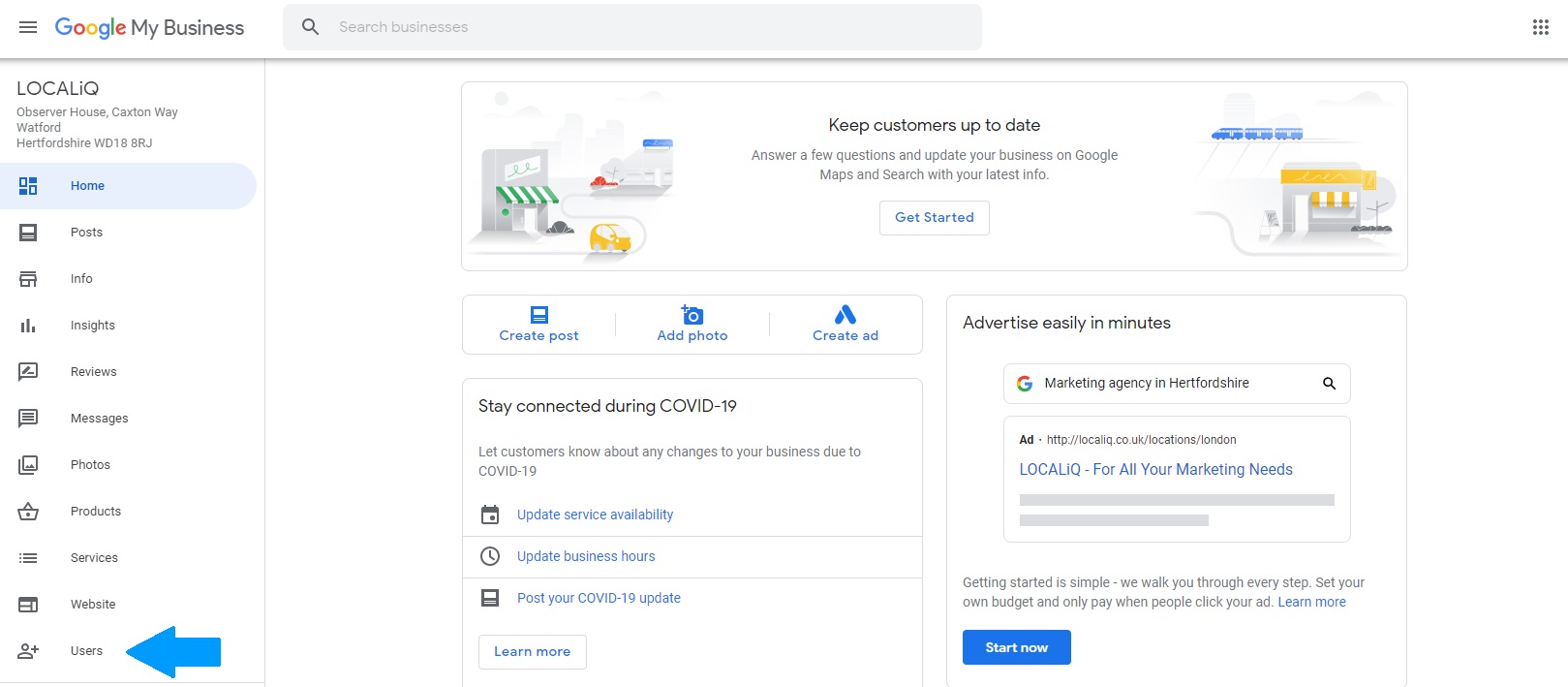This image is a detailed screenshot of a Google My Business dashboard. At the top left corner of the interface, "Google My Business" is prominently displayed. Adjacent to this label, on the right, is a gray search bar with the placeholder text "Search Businesses." Below this, on the left side, there is a vertical sidebar labeled "Local IQ."

The sidebar contains 11 navigational buttons, each featuring an icon to the left of their corresponding text. These buttons are ordered as follows: Home, Posts, Info, Insights, Reviews, Messages, Photos, Products, Services, Website, and Users.

On the main section of the dashboard, to the right, there is a highlighted header reading "Keep Customers Up to Date," accompanied by a prominent blue "Get Started" button situated directly below this message. Further down on the left-hand side, there are three blue buttons marked "Create Post," "Add Photo," and "Create Ad," each with a relevant icon above the text.

On the right side of the image, there's a section titled "Advertise Easily in Minutes," indicating an additional feature or tool available within the dashboard.